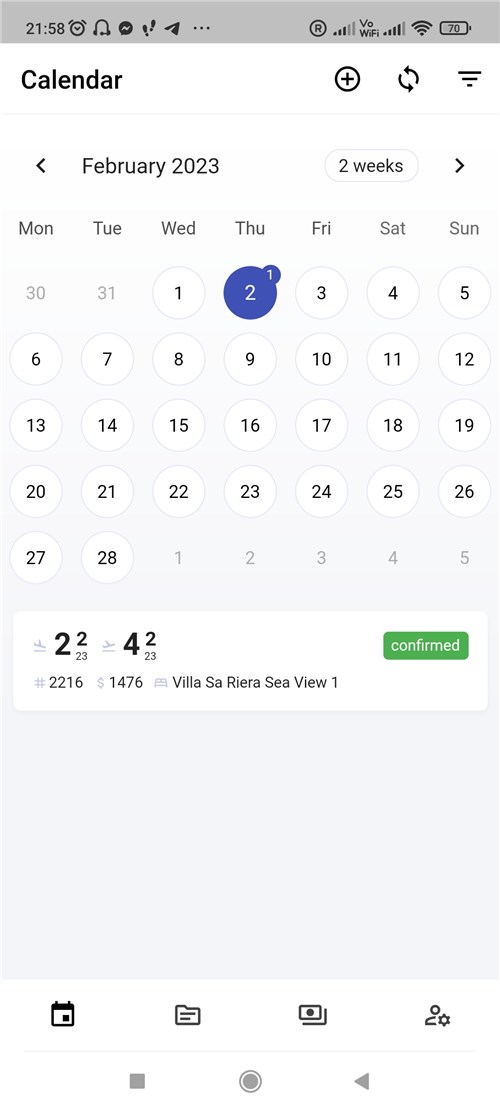This image is a screenshot from a mobile device showing the Calendar app interface. The background of the app is light gray, while the calendar itself appears on a white page. At the top-left corner of the screen, the word "Calendar" is displayed in black text. To the right of this, there are three icons: a plus symbol for adding events, a refresh symbol, and a list button.

The date displayed is February 2023, starting from Wednesday, the 1st, and ending on Tuesday, the 28th. The first Thursday, which is the 2nd, is highlighted in blue, indicating a scheduled event. Directly beneath the calendar grid, there is a confirmation of this event listed.